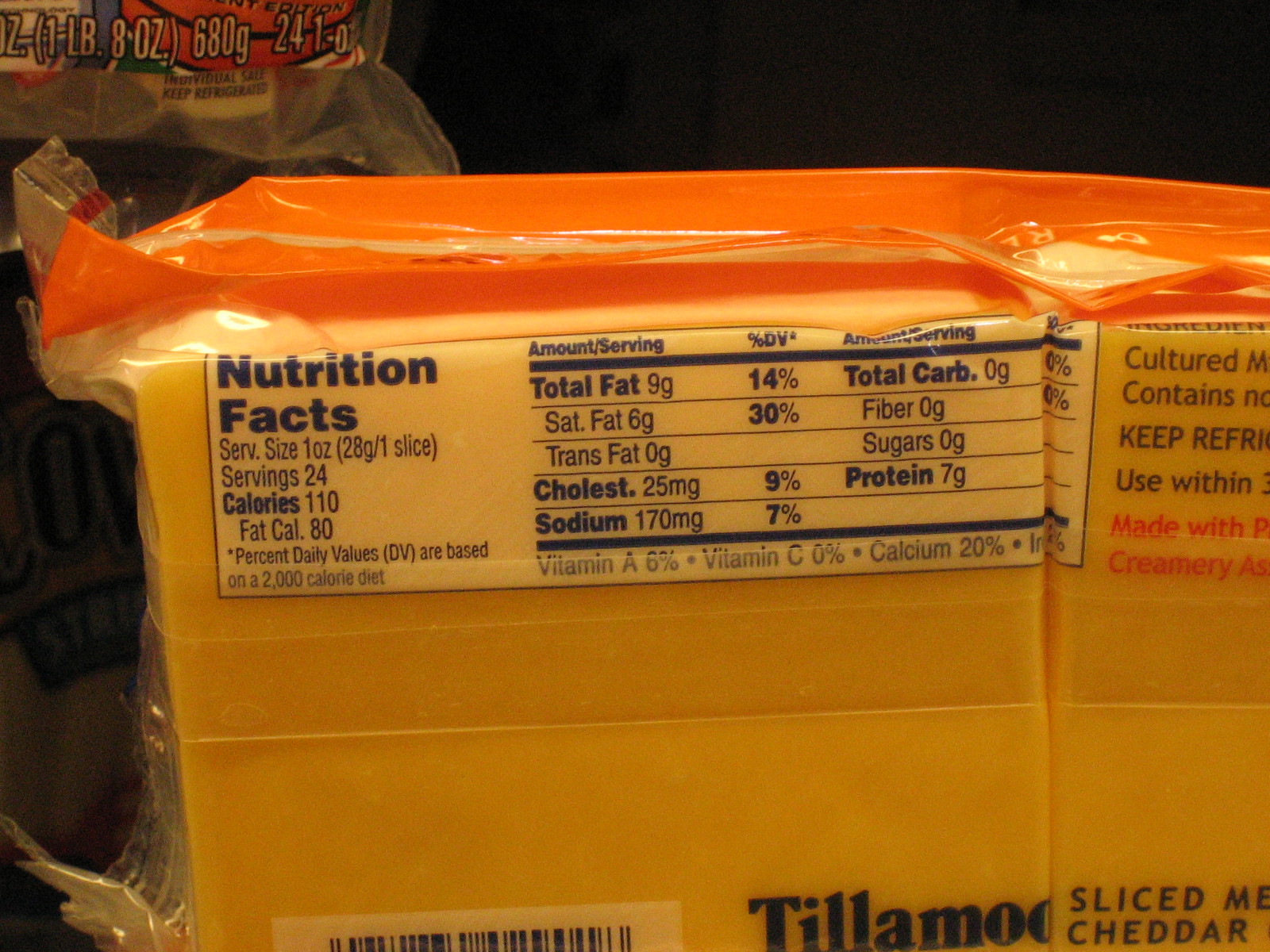This image displays a one-pound block of Tillamook Sliced Medium Cheddar Cheese, packaged in a clear wrapping with an orange seal at the top. The cheese's nutritional label is prominently featured, providing detailed nutritional information: each serving size is 1 ounce (28 grams), with a total of 24 servings. Each serving contains 110 calories, 80 of which are from fat. The label includes detailed breakdowns: total fat is 9 grams (14% daily value), saturated fat is 6 grams (30% daily value), cholesterol is 25 milligrams (9% daily value), sodium is 170 milligrams (7% daily value), and protein is 7 grams. It also lists vitamins and minerals: Vitamin A at 6%, Vitamin C at 0%, Calcium at 20%, and an indiscernible word that is likely iron. Part of the barcode is visible at the lower left of the package, and textual fragments indicating storage instructions are partially readable with phrases like "cultured," "contains," and "keep refrigerated." The label's text appears in black lettering against the clear packaging, which allows the light orange hue of the cheese to be visible. The cheese block is situated on what appears to be a table, and details such as “Medium Cheddar” are sliced into the cheese.